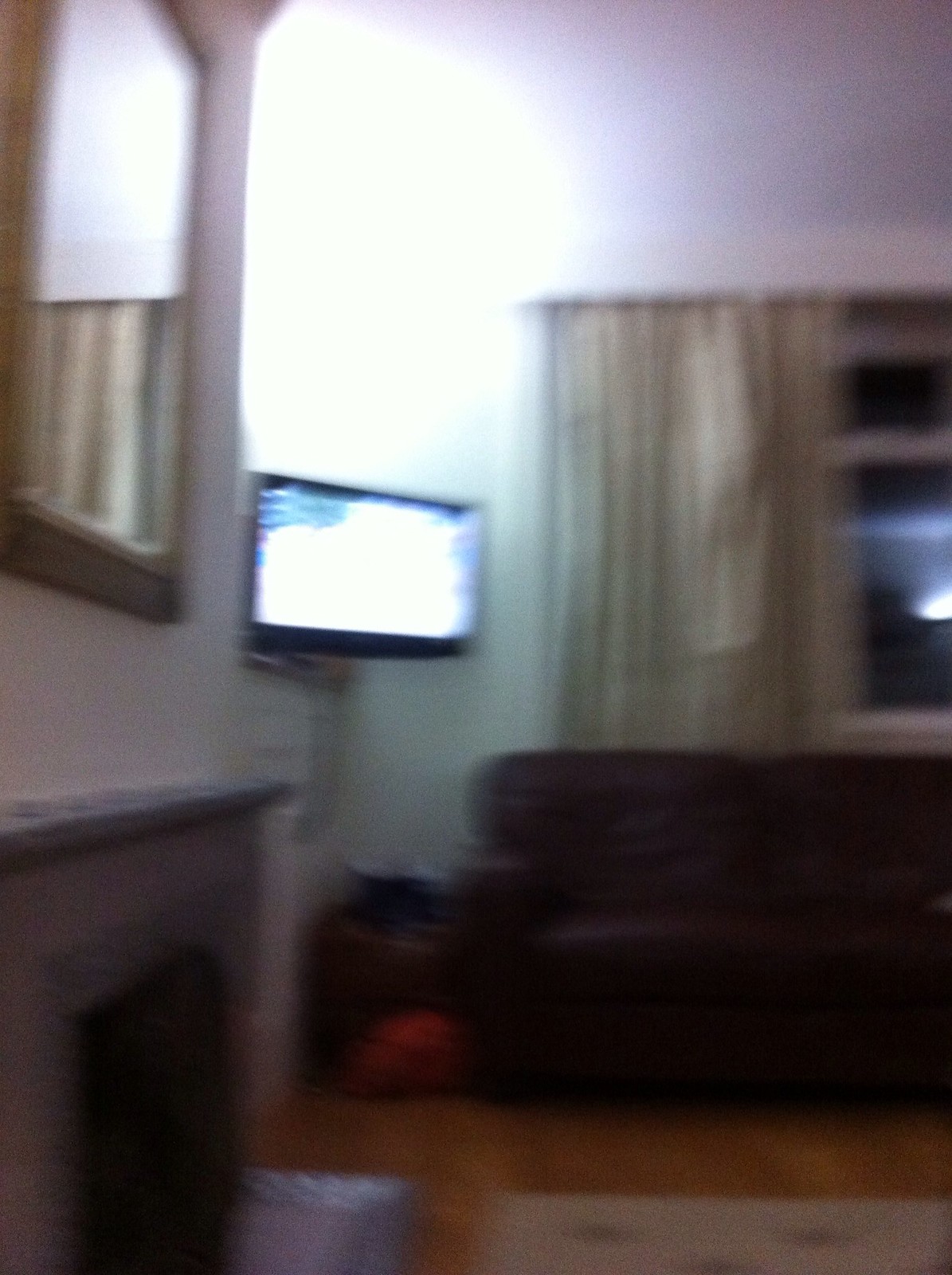This is a very blurry photograph of a living room taken during evening hours. The floor is a light hardwood with a barely visible beige carpet rug. To the left foreground, there is a whitish gray wall featuring a small fireplace with a mantle, above which hangs a mirror. The mirror reflects tan and white striped drapes that frame a closed window, indicating it is dark outside with no incoming light. A dark-colored sofa, possibly brown leather, is positioned against the far wall. In the corner between the window and the fireplace, a small television is mounted approximately four feet high, emitting a bright but indistinct image.